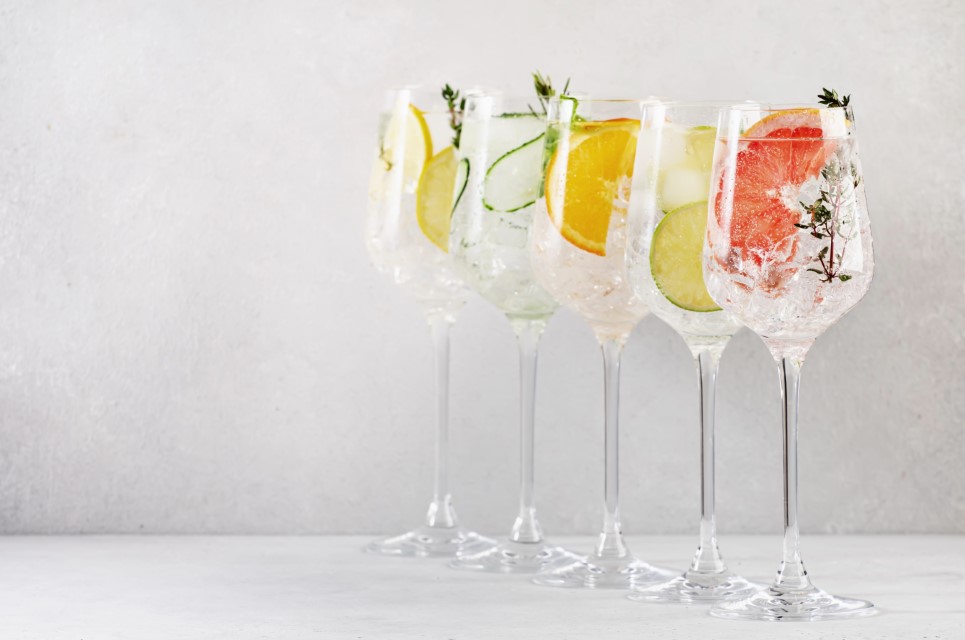This professionally-staged photograph, likely taken indoors, captures five crystal long-stem wine glasses arranged from left to right on a pristine white marble countertop, set against a textured gray wall. Each glass is filled with clear liquid, possibly water, and contains ice along with various garnishes. From the left to the right, the first glass features a lemon slice and a mint sprig; the second contains a cucumber slice and a mint sprig; the third includes an orange slice and a mint sprig; the fourth holds another mint sprig; and the closest glass on the right showcases a blood orange slice with a mint sprig. The professional lighting highlights the elegance and clarity of the composition, making this image both visually appealing and meticulously arranged, possibly for a luxury party or a high-end sale presentation.